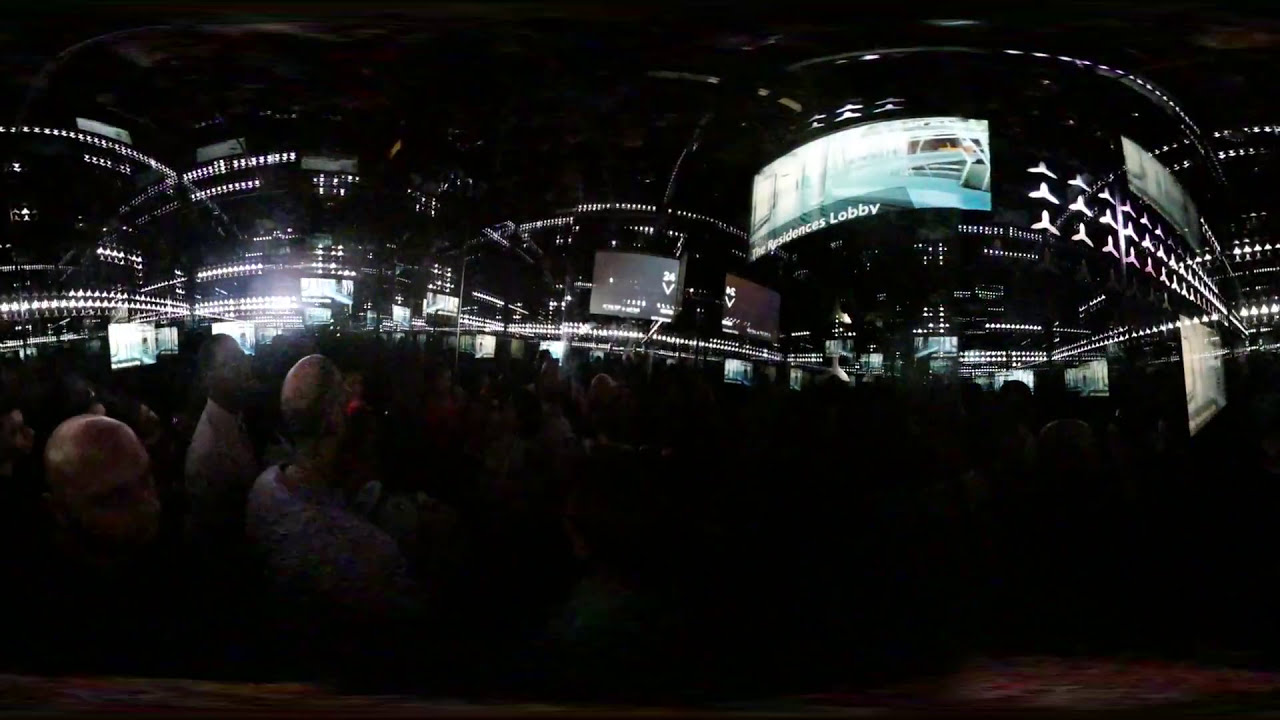In this captivating image, reminiscent of the bustling vibrancy of Times Square in New York City, we are presented with a dark, densely populated scene. The lower half of the image is dominated by a crowd of people, with some individuals more distinctly visible, such as a bald man and another with a receding hairline. The people are mostly seen as heads and silhouettes against a dark backdrop, giving a sense of an event or gathering. As our eyes move upward, the image brightens with an array of lights and billboards, creating a stark contrast with the dark foreground. 

Prominent among these illuminated displays is a large billboard featuring partially legible text, "Something Residences Lobby," although the full message remains unclear. The scene is awash with hues of black, white, various shades of gray, as well as splashes of blue, yellow, red, purple, and pink. The billboards and lights lend a futuristic vibe to the setting. Buildings frame the scene on the left, middle, and right sides, their facades brightly lit and contributing to the overall dazzling effect. 

This unique and energetic depiction captures the essence of a major city's nightlife, where people gather, interact, and immerse themselves in the electric atmosphere of light and color.